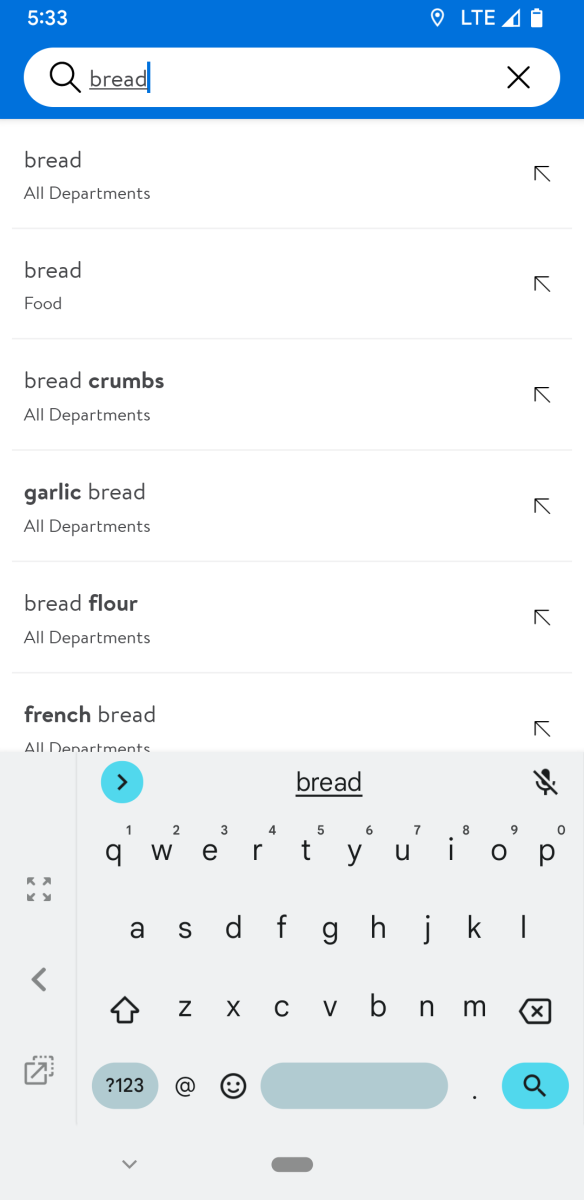A screenshot of an Android device showcases the screen at 5:33 AM, as indicated by the time displayed in the top-left corner. On the top-right corner, various status icons are visible, including the location status, network signal strength, LTE connectivity, and the battery level indicator. Dominating the screen is a search box with the input text "bread," triggering a list of search results. These results include categories such as "bread - all departments," "bread - food," "breadcrumbs - all departments," "garlic bread - all departments," "bread flour - all departments," and "French bread." Beneath the search results, the phone's virtual keyboard is partially visible, ready for further user input.